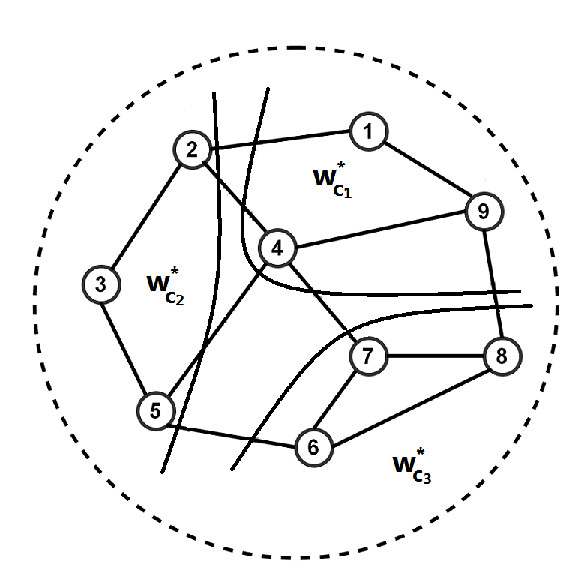This image showcases a detailed diagram that seems to relate to a mathematical problem or perhaps a complex riddle. At its core, the diagram features an octagonal shape, enclosed within a dotted line circle. Each of the eight corners of the octagon is numbered, along with several lines crisscrossing its interior, creating intersections that are also labeled. There are a total of nine intersections marked from 1 to 9. 

Intricately drawn within this octagonal figure are parabola-like curves, resembling hills or arcs, that traverse the interior at various angles. In addition to this, the diagram is segmented into three distinct fields or sections labeled W * C1, W * C2, and W * C3. Notably, W * C1 and W * C2 are positioned inside the octagon, whereas W * C3 resides in the space between the octagon and the surrounding circle. This detailed layout appears meticulously organized, suggesting a structured approach to solving or explaining a complex concept.